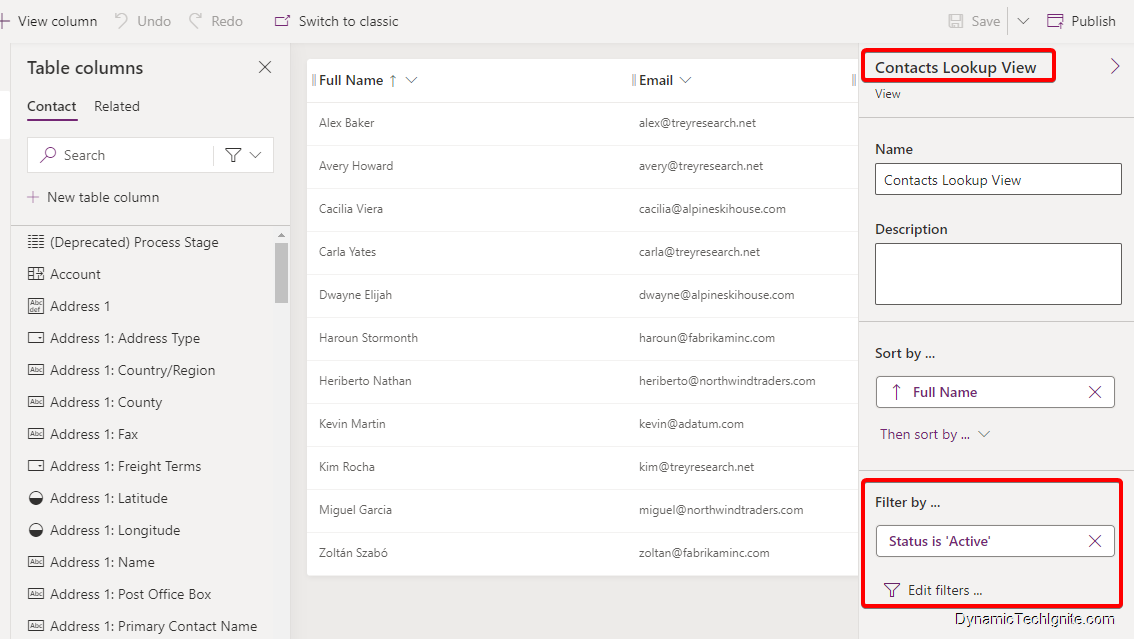The screenshot captures a web interface with several highlighted areas. At the top of the screen, there are options labeled "View Column," "Undo," "Redo," and a button for "Switch to Classic." The left sidebar features a section titled "Table Columns," with subsections for "Contact" and "Related," the former underlined with a purple line. Below that, there is a search bar and a button for adding a new table column. The sidebar continues with multiple icons and options for various addresses, such as "Address 1" and "Address for this," each clickable for further actions.

In the center of the screen, a rectangular section is divided into two columns: the left column lists a person's full name, while the right column displays their email address. To the far right, there is a marked section labeled "Contacts Lookup View," outlined with a bold red rectangle. At the bottom of the screen, another area labeled "Filter By" is also highlighted with a red border, directing attention to it. These prominent red outlines emphasize important sections within the interface for easy navigation and clarity.